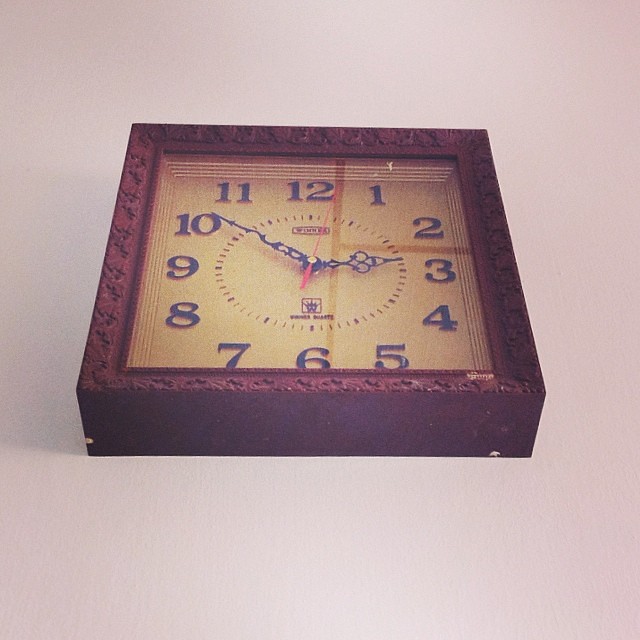This photograph captures a vintage square clock, positioned diagonally on an off-white surface, providing a partial view of both its face and base. The clock is made of wood, featuring an intricately carved, ornate frame that resembles a deep picture frame. The face of the clock, covered with glass or plastic, is beige or cream-colored, adorned with black, decorative hands and a red second hand. The numbers 1 through 12 are clearly displayed, and small dashes mark each minute. A noticeable brown line extends vertically just to the right of the 12 and 6, with another line branching toward the right above the 3. The time indicated is approximately eight or nine minutes until three, set against a backdrop that casts subtle shadows, adding depth to the scene.